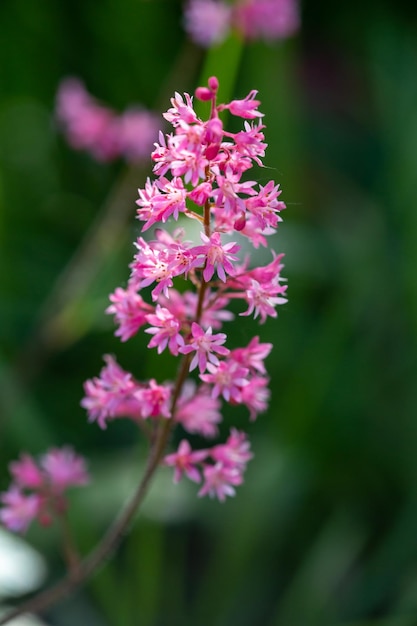The image is a detailed color photograph in portrait orientation, showcasing a flowering plant as its main subject. The background is an out-of-focus blend of dark green hues, with lighter green areas that might resemble blurred blades of grass, and a few scattered pink flowers. Emerging from the bottom left corner, a dark greenish-brown stem arcs gracefully towards the center and then vertically upwards. Clusters of small pink flowers, numbering around 50, adorn this stem. Most flowers feature a yellowish center, creating a dotted appearance, and are interspersed with unopened pink buds near the top. While the lower blossoms are slightly blurred, those near the top are in sharper focus, revealing more detail. The overall effect is a branch laden with pink flowers and buds, contrasted against a green, impressionistic backdrop.